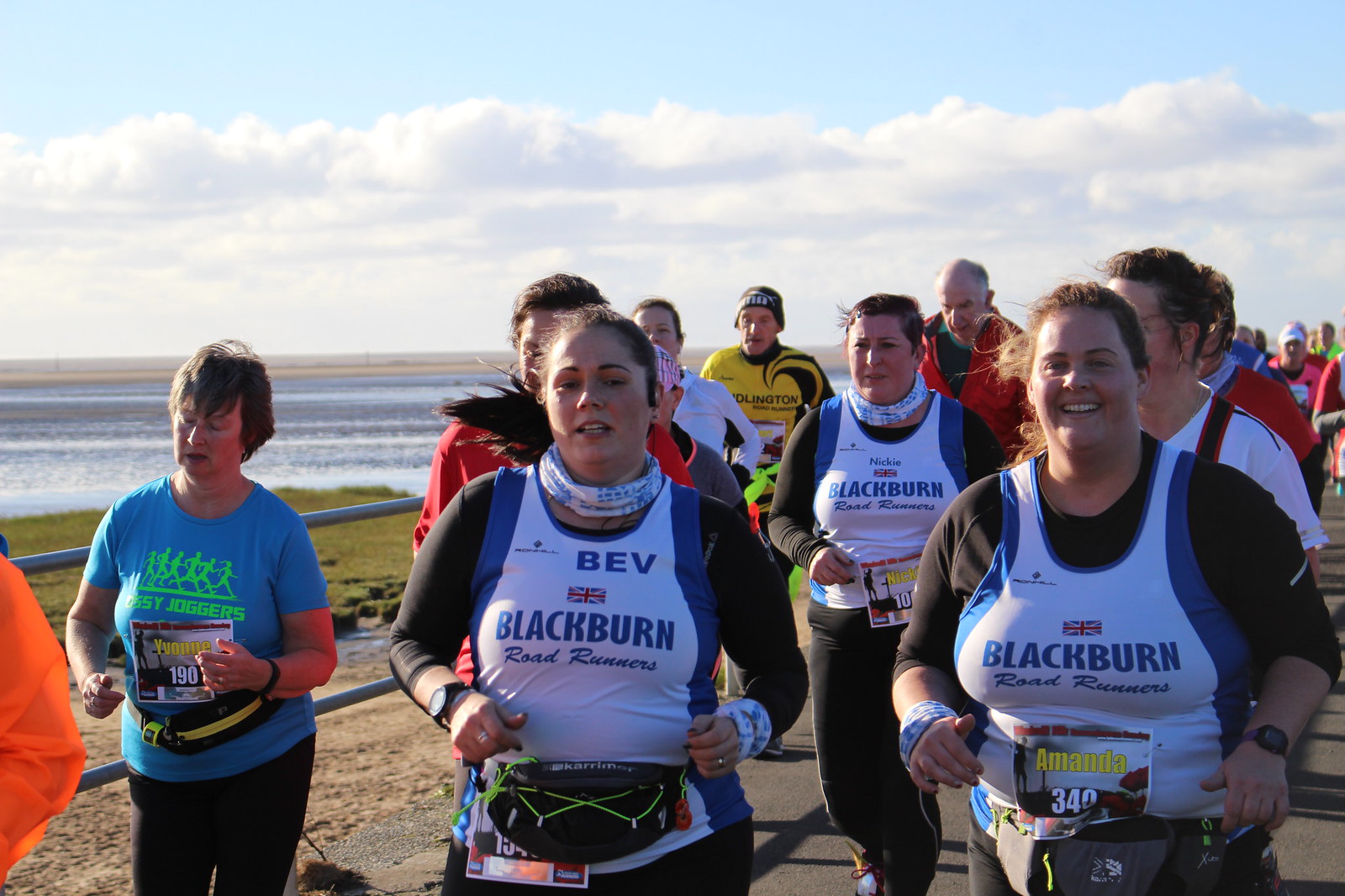The image captures a lively outdoor running event on a sunny day with a light blue sky scattered with dark and white clouds. In the foreground, a diverse group of men and women are jogging along a path by the water, which appears to be a large lake or ocean, separated from the runners by a gray metal railing. Among them, three women in the front draw attention by wearing coordinated outfits—white tank tops with blue sides, black long-sleeve shirts underneath, and “Blackburn Roadrunners” emblazoned in blue text, complete with small UK flags. One of these shirts reads “Bev,” another “Nikki,” while the third remains unnamed. Alongside them is a woman in a light blue shirt with a neon gray graphic labeled "Bossy Joggers," bearing the race number 190. In total, at least 14 participants, ranging in attire and body type, can be seen running at a steady pace, adding a sense of camaraderie and activity to the serene beachside landscape.